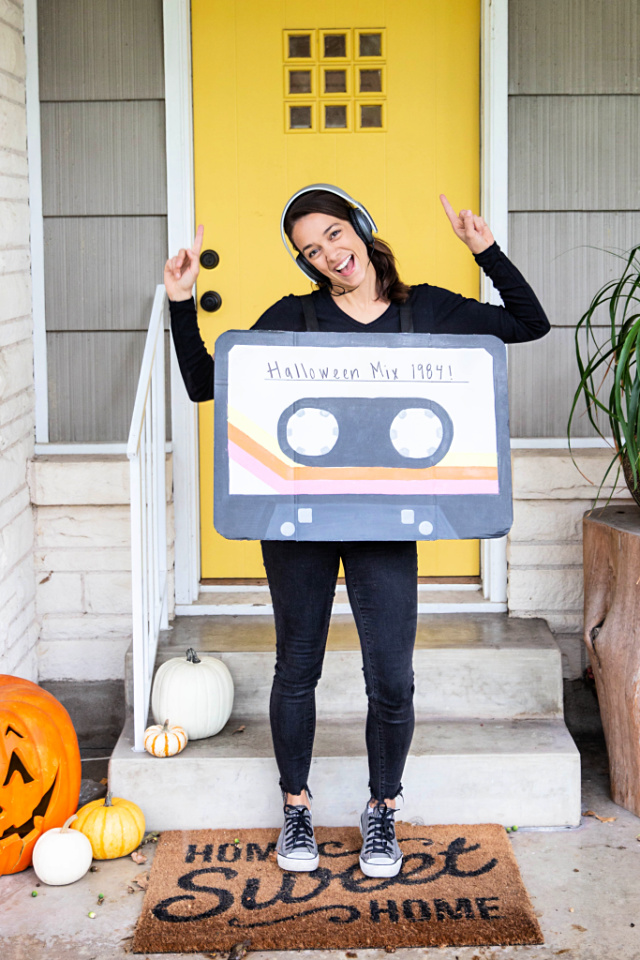In this charming family photograph, a woman stands outside her front door, gleefully dressed as a cassette tape for Halloween. Her costume features a cardboard replica of a black cassette tape, adorned with a white label that reads "Halloween Mix 1984" and is decorated with pink and orange diagonal stripes at the bottom. She wears headphones and complements her costume with a black long-sleeved shirt, black jeans, and stylish gray Converse sneakers. The woman has her arms raised with her index fingers pointed upwards, exuding playful energy.

She stands on a brown and black doormat inscribed with "Home Sweet Home," surrounded by seasonal decorations. Behind her, the front door, painted a vibrant yellow and adorned with nine glass inserts, opens into an off-gray house. To her left, a white railing frames the scene, while a variety of pumpkins cascade across the concrete steps. A white pumpkin and a smaller striped one sit on the first step, while an orange pumpkin, another white pumpkin, and a carved jack-o'-lantern rest near the bottom. A green plant adds a touch of life on her right. This photograph captures the quintessential Halloween spirit and the warmth of home.